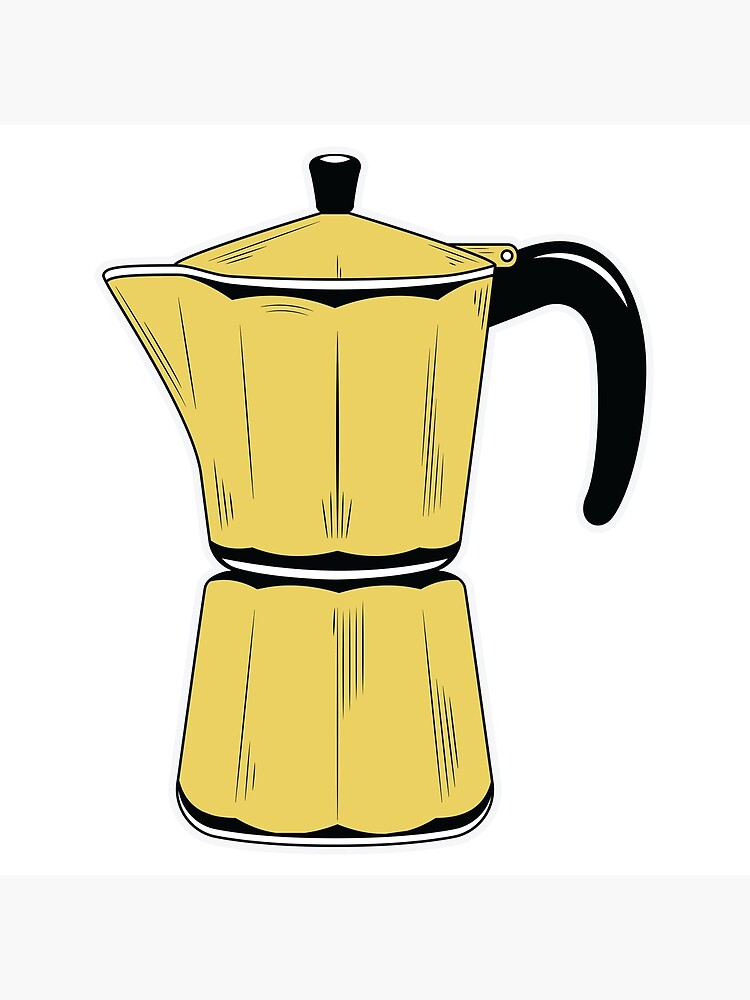This is a simple, clean graphic drawing of a yellow teapot, or possible espresso maker, featuring a curved black handle on the right side and a black knob on the yellow lid. The teapot sits on a long cylindrical cup of the same pastel yellow color, identical in style and adorned with a black and white border at the bottom. The top of the teapot has a small spout for pouring, and the entire image is set against a primarily white background with gray borders above and below. The detailed lines illustrate the separations and contours of the teapot and cup, enhancing the clarity and classical aesthetic of the overall design.